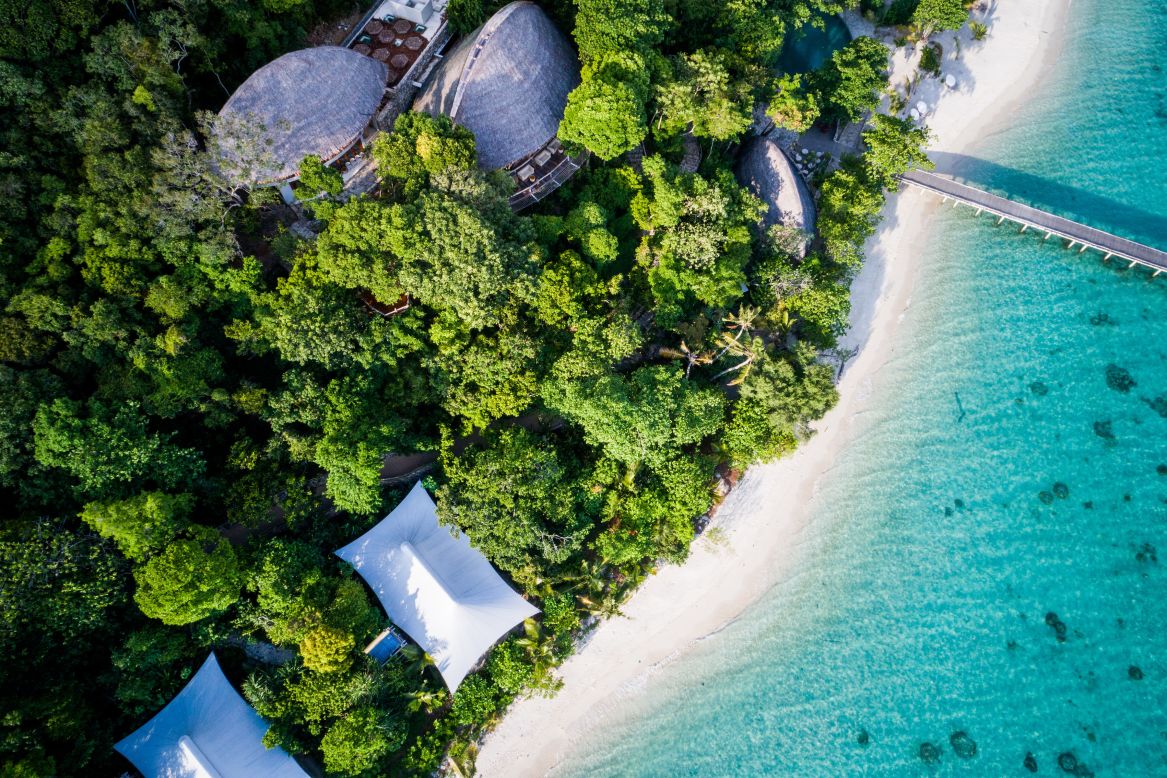This image captures an aerial view of a vibrant beachfront landscape. From above, the scene showcases a dense wooded area filled with bright green trees that extend up to the edge of a pristine white sand beach. Nestled within the trees are two prominent square roofs, likely belonging to high-end homes or resort buildings, partially white in color with hints of light blue, suggesting perhaps decorative elements or open-air spaces like balconies with seating. Additionally, a more rounded roof structure can be seen among the trees, possibly indicative of a gazebo or another recreational facility. The beach itself transitions into crystal-clear blue waters where underwater plants and other marine features are visible. A bridge or small roadway connects the verdant forested area to another unspecified region beyond the image's scope, hinting at further exploration. The clarity of the water reveals the presence of dark, rock-like formations just below the surface, adding to the natural allure of the coastal setting. The entire scene is bathed in natural light, emphasizing the contrast between the lush greenery, the bright beach, and the inviting waters, encapsulating a picturesque and serene coastal haven.